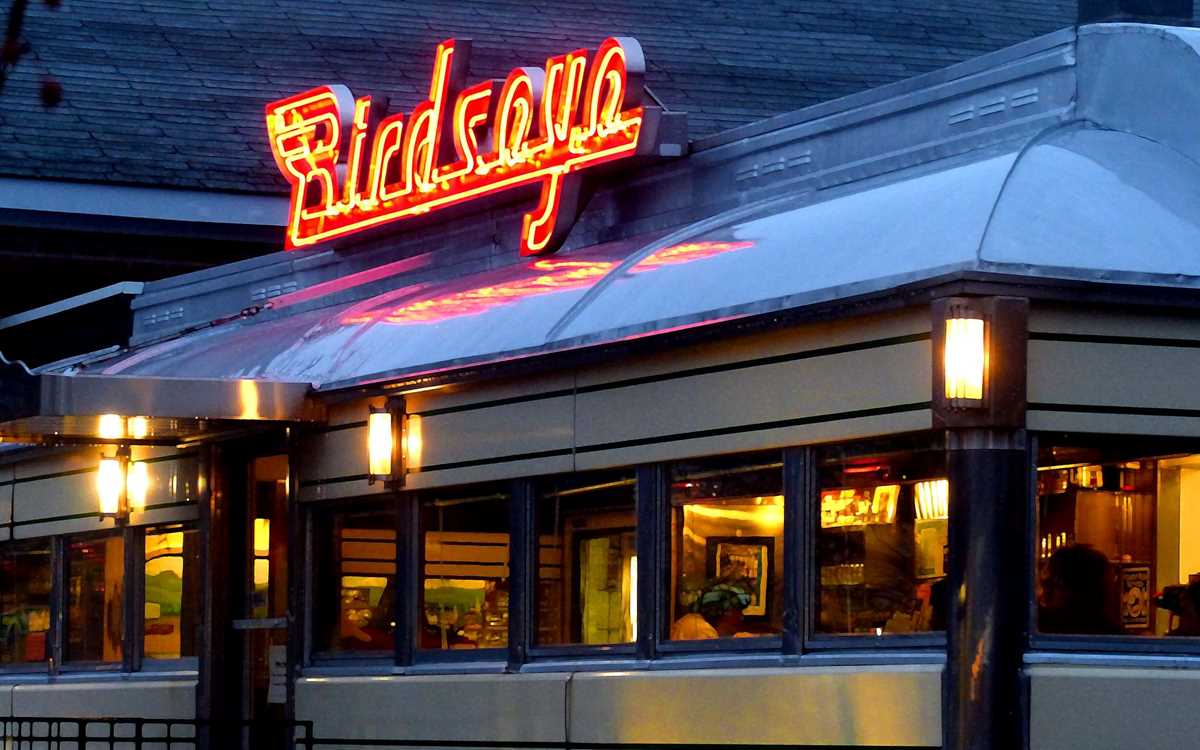This image showcases a diner reminiscent of a vintage train car or bus, with a rounded top and a shiny silver exterior. The scene is set at dusk, with the soft glow of outdoor lights beginning to illuminate the surroundings. Prominently displayed atop the midsection of the roof is an eye-catching sign that reads "Birdseye" in bold, red fluorescent letters accented with bright yellow, creating a vibrant and welcoming atmosphere. Through the large square windows, the dimly lit interior reveals patrons enjoying their meals, including a man wearing a green hat and an orange shirt. The overall composition and lighting suggest this professional photo might be used to promote the nostalgic charm and inviting ambiance of the diner.